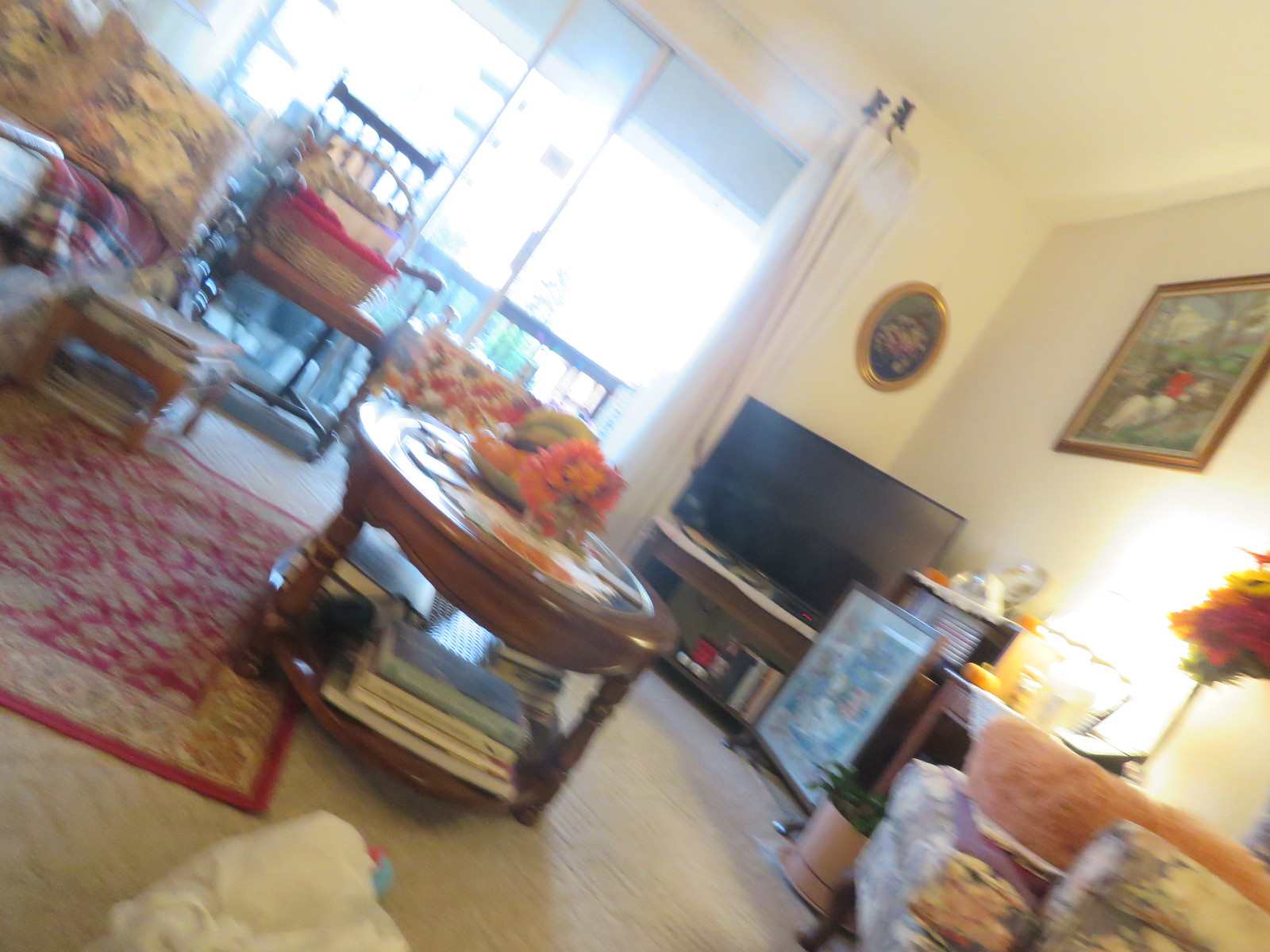This slightly tilted and blurry indoor color photograph captures a well-lit living room, primarily illuminated by a large window that allows ample natural light. Positioned in the back of the room is a patio door, seemingly open, which complements the room’s bright atmosphere. On the right side, there is a credenza with a large flat-panel TV situated in the corner. Above the TV, a mounted oval artwork is noticeable, and further to the right, a square framed picture hangs on the white wall, accentuated by a lit lamp beneath it.

To the left, we see a rocking chair near another framed photo. Dominating the central space is a round wooden coffee table, adorned with a fall-themed centerpiece and additional books on its lower shelf. The flooring is carpeted in light tan, with part of an area rug visible near the coffee table. A couch filled with large, flower-printed pillows is positioned in the upper left corner.

The living room setup hints at cozy, lived-in vibes with strategically placed furniture, including an additional seat near the right side and decorative elements such as a photo frame, giving the room a touch of personality. Despite the image’s lack of focus and its slightly slanted perspective, it encapsulates a warm, welcoming living area within an apartment building.